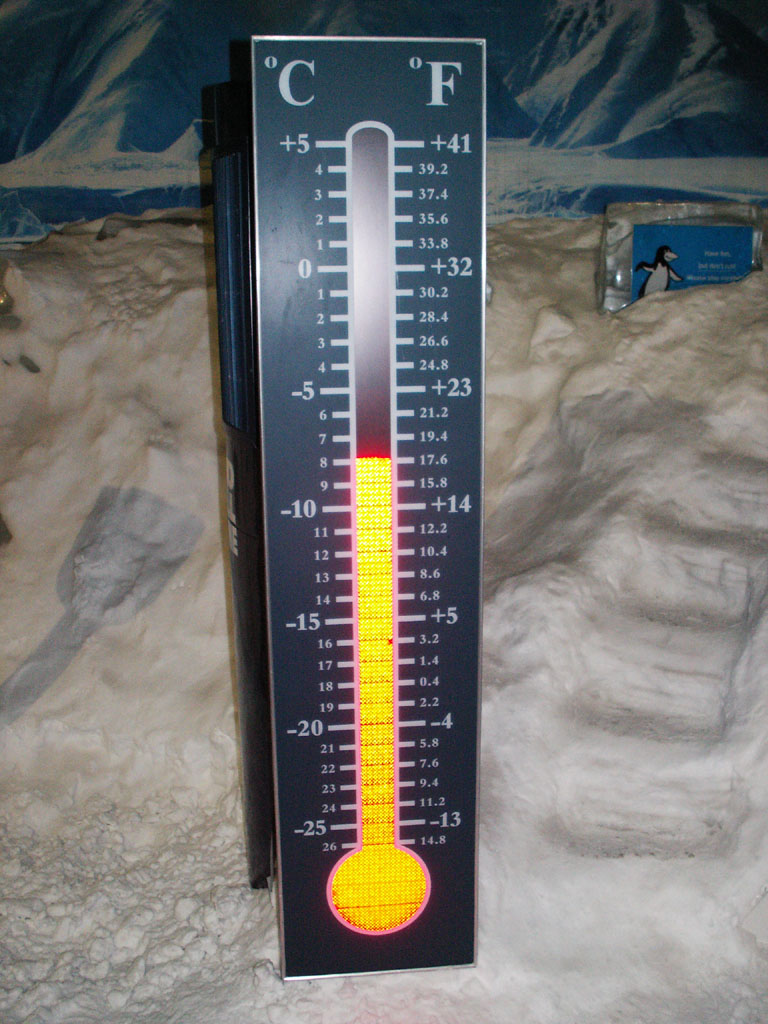The image prominently features a long, rectangular thermometer set against an intricate and detailed background designed to evoke a penguin habitat. The thermometer itself is navy blue, with a curved, rounded top that runs the length of the instrument, and it's marked with temperature graduations in both Celsius and Fahrenheit. On the left side, Celsius degrees range from +5°C down to -26°C, with detailed markings at each degree and larger numerals at intervals of five. The right side shows Fahrenheit degrees, ranging from +41°F down to -14.8°F, presenting similar detailed markings and larger numerals at specific intervals.

The central part of the thermometer, which houses the yellow mercury tube, indicates a temperature of approximately -8°C or 17.6°F. The tube extends along the entire instrument, culminating in a larger circle at the bottom.

In the background, the scene is crafted to simulate a penguin habitat, characterized by fake snow and ice. A small, carved staircase ascends through the artificial snowy hills, adding to the illusion of a chilly Arctic environment. Further contributing to this effect, the backdrop showcases a painted image of snowy mountains and glaciers in shades of white and blue. 

On the right side of the background, there's a small cartoon-like penguin with white text that is unreadable, placed against a blue backdrop and affixed to a faux stone. The overall scene is meticulously designed to replicate a cold, wintry landscape, creating a fitting context for the thermometer's placement.